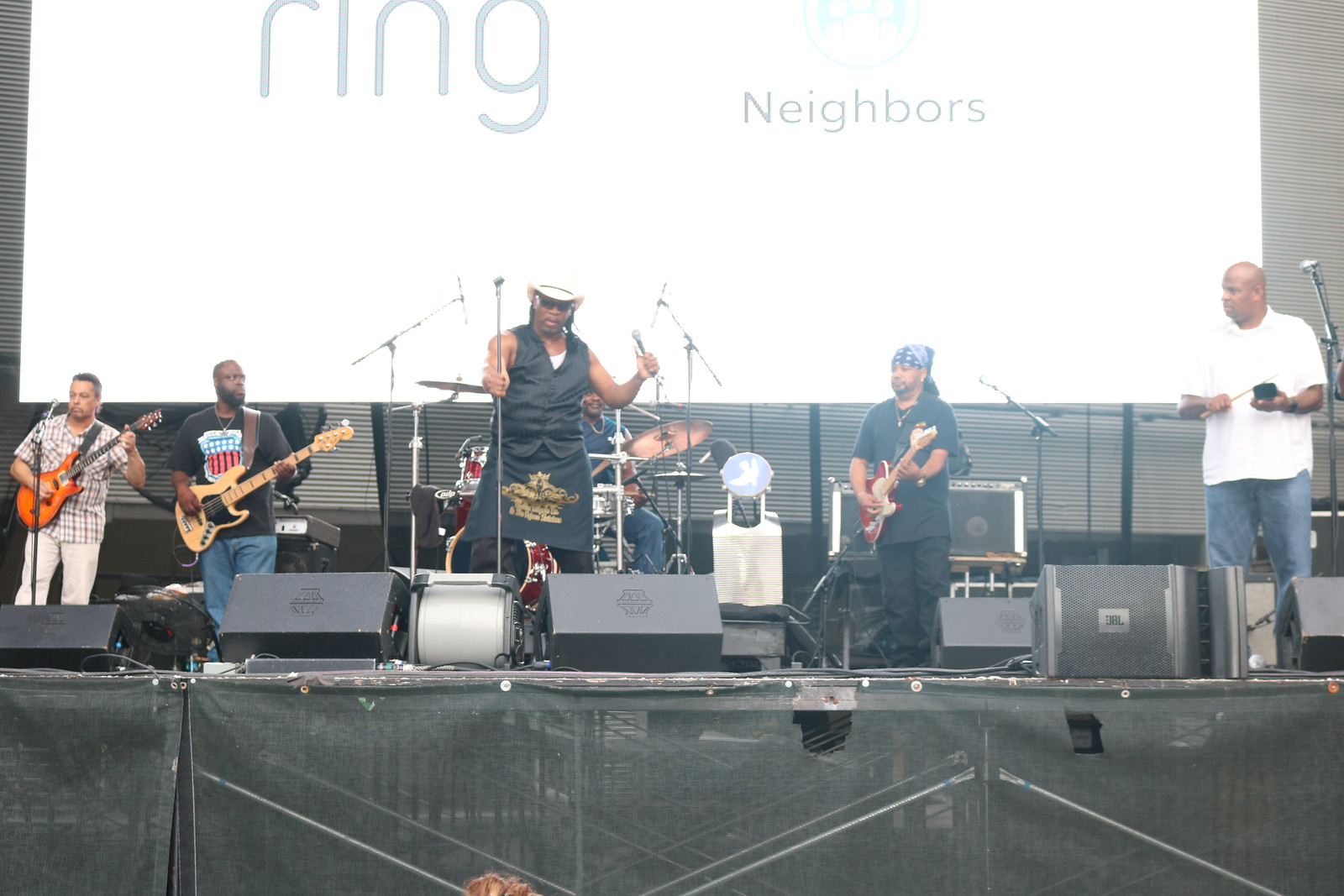This photograph captures a lively stage performance by a six-member band, prominently featuring a diverse ensemble of musicians. Center stage is the lead singer, a darker-skinned African American man adorned in dark glasses, a white cowboy hat, a black vest over a white shirt, and a distinctive black and gold skirt. He holds a microphone, engaging with the audience. The backdrop behind him displays the words "Ring Neighbors" in a blueprint-like design, partially obscured by a symbol, all set against a white screen with gray sides. 

Flanking the lead singer are three guitarists: to the left, a white man in an all-white outfit playing a brown guitar, and next to him, an African American man in a black t-shirt and jeans, sporting a red and blue emblem, and strumming a tan and black guitar. To the right, another guitarist, likely African American, is distinguished by a do-rag (possibly blue or black), long hair, and an all-black outfit, playing a red and white guitar. On the far right stands a tall, bald African American man in a white dress shirt and blue jeans, playing an unidentified small black instrument with a brown drumstick. 

Behind the lead singer are drummers, one with a vivid red drum set, contributing rhythm to the ensemble. The front of the stage is equipped with speakers and cables, while a black cloth drapes the bottom, adding to the concert ambiance. The gray and black tones of the background walls enhance the overall aesthetic, indicating a possible live gig given the visible heads of audience members.